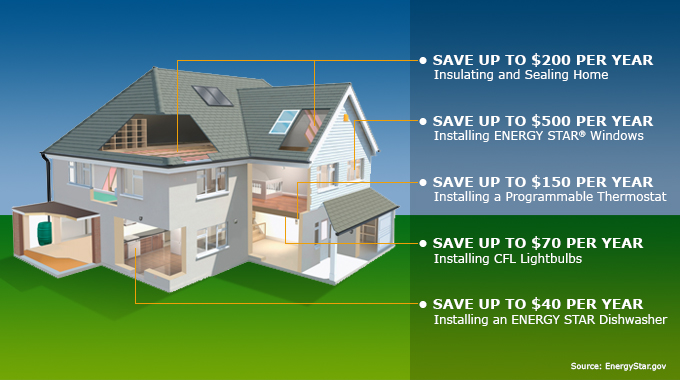The illustration details how implementing energy efficiency measures can save on household expenses. The image, set against a blue sky and green lawn background, features a two-story house with sections of the roof and walls cut away to reveal the interior, including the loft, kitchen, porch, and garage. Surrounding the house are five arrows indicating potential yearly savings from different upgrades: up to £200 by insulating and sealing the home, $500 by installing ENERGY STAR windows, $150 by using a programmable thermostat, $70 by switching to CFL light bulbs, and $40 by installing an ENERGY STAR dishwasher. To the right, corresponding bullet points provide these savings figures, and at the bottom right, in small text, the source is cited as energy star dot gov.